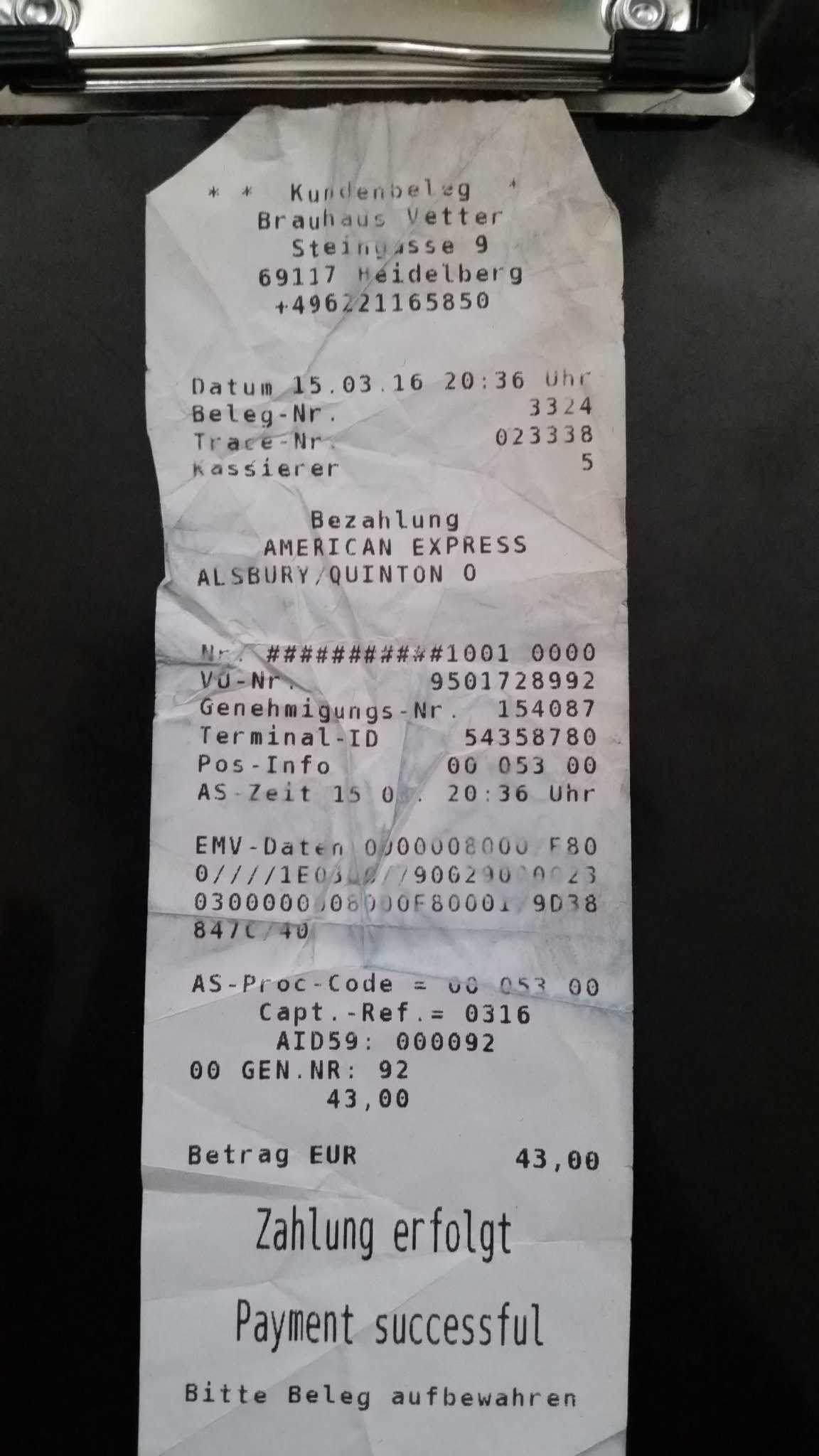The image depicts a worn, slightly faded receipt that is firmly clamped to the top of a clipboard, identifiable by a metallic silver bar designed to secure papers. The receipt, which appears to have been through some wear and tear, is filled with various small numbers printed in black ink. Prominently displayed in the middle at the top is the header "Besalung American Express," followed by the name "Ellsberg, Quinton, Ohio." A contact number, 496-211-6580, is also present at the top. Although the address printed below is partially faded and difficult to read, it is still somewhat visible. At the very bottom of the receipt, the phrase "Zalong Earth Folgates payment successful" is clearly printed, confirming the completion of a transaction. The receipt and clipboard are set against a solid black background, highlighting the aged and crumpled texture of the paper.